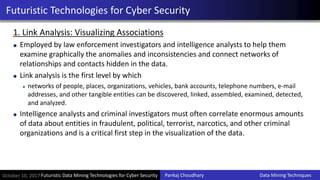The image is a compressed, small screenshot of a PowerPoint slide titled "Futuristic Technologies for Cybersecurity," set against a basic white background with a blue trim at the top and bottom. The title is displayed in white text within a blue and black rectangle at the top. The main body of the slide contains extensive black text that is difficult to read due to the image's low resolution. However, it lists "1. Link Analysis: Visualizing Associations," followed by three detailed bullet points. The first bullet point explains that link analysis is employed by law enforcement investigators and intelligence analysts to graphically examine anomalies, inconsistencies, and networks of hidden relationships and contacts in data. The second bullet point describes link analysis as a method for discovering, linking, assembling, examining, detecting, and analyzing networks of people, places, organizations, vehicles, bank accounts, telephone numbers, emails, addresses, and other tangible entities. The third bullet point emphasizes that correlating vast amounts of data about entities involved in fraudulent, political, terrorist, narcotics, and other criminal organizations is a crucial first step in data visualization for intelligence analysts and criminal investigators.